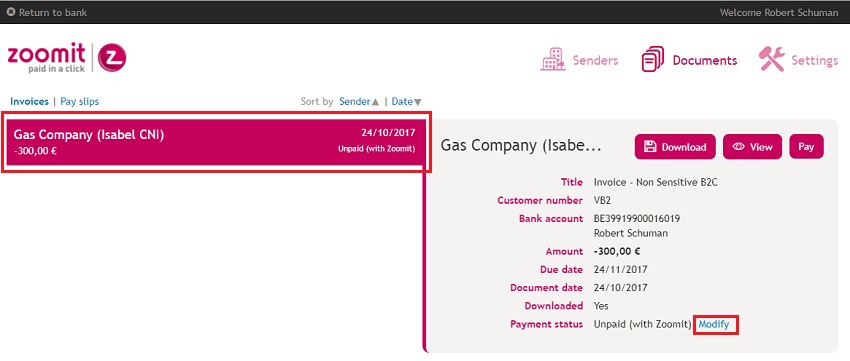The screenshot displays an online banking invoice interface. At the top of the screen, there is a black border with the text "Welcome Robert Schuman" written in gray on the top right. On the top left, there is an "X" button situated next to a "Return to Bank" button.

Centrally, the interface features "Zoomit" branding, with the text "Zoomit, paid in a click" in pink. A pink circle with a white "Z" logo is positioned next to this text. To the right of the logo, navigational links "Senders," "Documents," and "Settings" are also in pink font. 

The section below features blue font with labels for "Invoices," "Payslips," and sorting options by "Sender" and "Date." There is a prominent red box highlighting an invoice section that provides information about a gas company bill.

Within this red box, the invoice details are as follows:
- Sender: Gas Company, Isabel
- Customer Number: VB2
- CNI: (identifier) minus 300 Euro
- Invoice Date: 24-10-2017
- Document Type: Non-Sensitive, B2C
- Bank Account: BE399-199-000-16019
- Billed To: Robert Schuman
- Invoice Amount: -300 Euros
- Due Date: 24-11-2017
- Payment Status: Unpaid with Zoomit
- Downloaded: Yes

On the right-hand side within the same red box, options to download, view, or pay the invoice are available, labeled as "Download," "View," "Pay." These labels are in gray, along with invoice details and the "Modify" button which is highlighted in blue and also boxed in red.